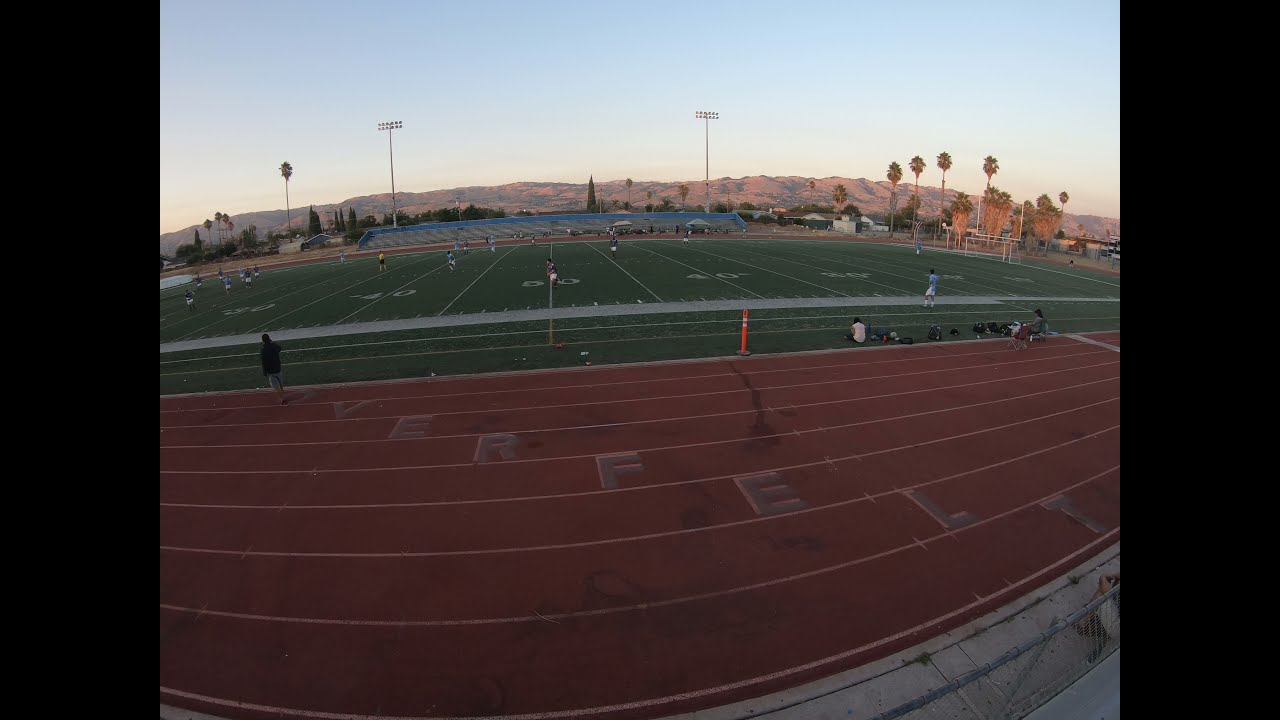The photograph captures an athletic field featuring a red running track encircling a green football field marked with white yard lines, such as 50-yard, 40-yard, 60, 70, and 80. Prominently displayed on the track are the faintly visible letters "OVERFELT." Multiple individuals are present: one wearing a dark jacket is standing on the track, another is walking on the left side, and several are gathered around the field's edges, presumably watching a game. In the background, small figures of players clad in blue, white, and yellow uniforms can be seen on the field. Further back, spectators are seated in bleachers, with the scene framed by brown hills, palm trees, and tall stadium lights under a hazy blue sky.